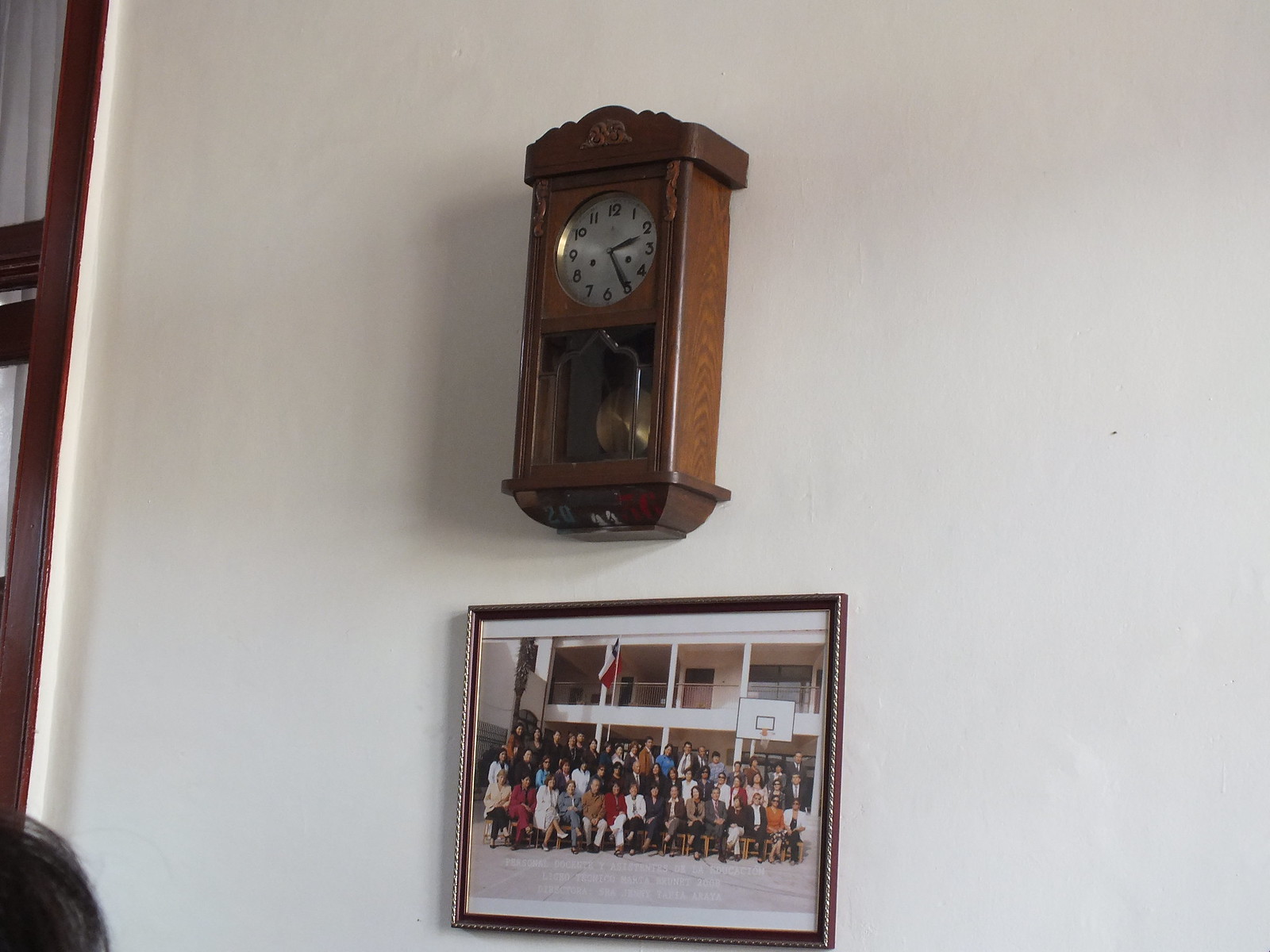The photograph captures a white wall in a house, prominently featuring a dark brown, wooden grandfather-style clock and a framed group photo arranged vertically. The clock, mounted above the picture, boasts a long rectangular wooden body with a brass pendulum visible through a glass window in its lower half. The circular clock face, set against the wooden frame, displays black numbers from 1 to 12, and reads 2:25. The clock’s design is reminiscent of a cuckoo clock, with a thick wooden frame and a golden pendulum that swings below the glass section.

Directly beneath the clock is a silvery, squarish picture frame, slightly larger than A5 size, containing a large group photo. This appears to be a class or staff photo with three rows of people: the front row seated on stools, the middle row standing, and the back row elevated, possibly on stools. The group is posed in front of a two-story building featuring a flag and a basketball hoop attached to its balcony. The image conveys a sense of nostalgia and communal memory, captured in the timeless contrast between the antique clock and the formal group photograph.